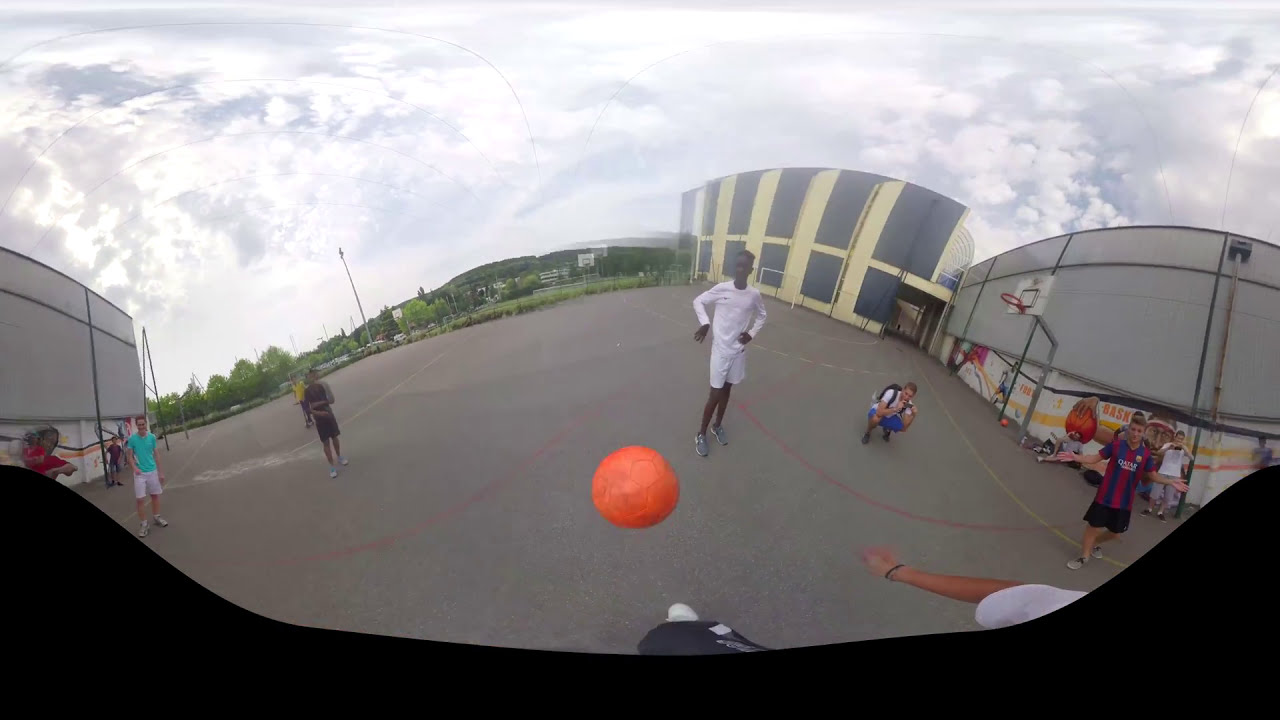In this detailed image, a variety of kids are playing soccer on a gray asphalt or concrete parking lot, marked with red, yellow, and white lines. The scene is captured from a first-person perspective, likely from a camera mounted on someone's head or helmet, depicting an action-packed moment as an orange soccer ball is about to be kicked by someone in black pants, white shoes, and a white shirt with black rubber bands around the wrists. The bustling environment reveals multiple players spread across the lot. On the left side, one can notice kids wearing a mix of green, white, black, yellow, blue, and red attire, while on the right side, beside the central ball-kicker, there’s a kid in all white and another crouching with a black backpack, white t-shirt, and blue shorts. Nearby, another kid throws out his arms in a blue and red striped shirt with black shorts, accompanied by a kid in a white shirt. In the backdrop, framed by a cloudy sky with thick white clouds, stands a school building adorned with a mural in yellow and blue stripes featuring a painted figure, alongside a basketball hoop, and further structures partially obscured by green trees. The overall ambiance indicates an outdoor setting in the middle of the day, showcasing an energetic game of soccer amidst a lively schoolyard scene.